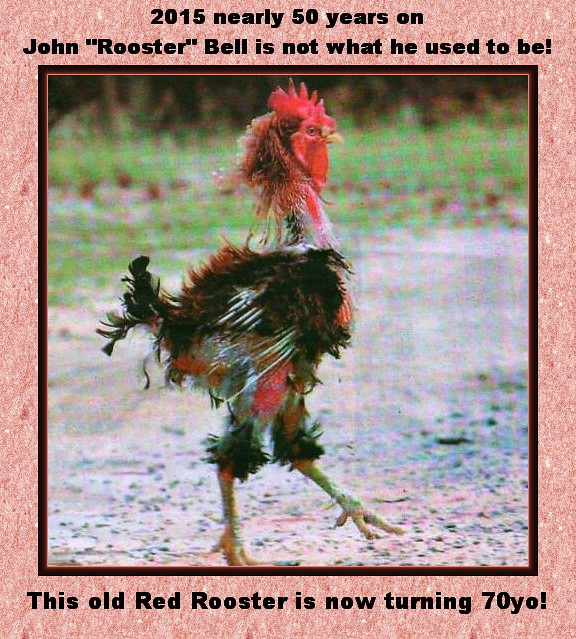The image features a close-up photograph of an old, decrepit rooster named John Rooster Bell, situated in the center of the frame. The rooster has lost a considerable amount of feathers and appears unhealthy, with unruly dark brown to black plumage, a red head, a yellow beak, and yellow claws. The rooster is captured in side profile, moving from left to right across a dirt and rocky ground. The background is out of focus, showing hints of grass and bushes.

The photograph is bordered by a black frame, set on a rose-colored surface with a marbled texture. Above the image, text in black font reads, "2015, nearly 50 years on. John Rooster Bell is not what he used to be." At the bottom, the text continues, "This old rooster is now turning 70 years old!" The overall presentation appears to be a nostalgic birthday greeting card for the aging rooster.